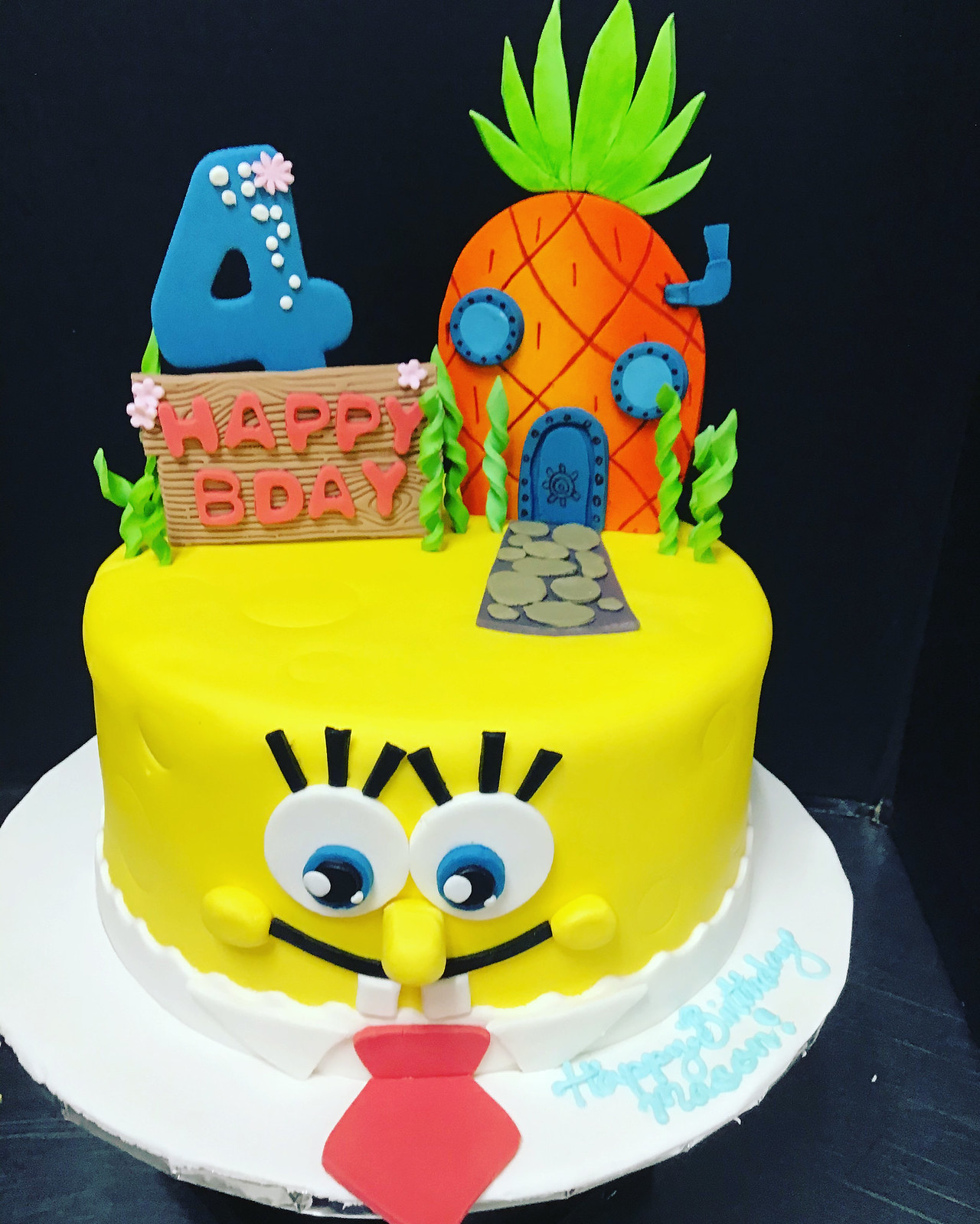This image depicts a highly detailed, cartoon-style birthday cake themed after Spongebob Squarepants, set against a black background. The cake, which takes up most of the image, is placed on a white plate or cardboard disk. Scripted in light blue icing on the disk are the words "Happy Birthday" followed by an illegible name. The main body of the cake is coated in bright yellow fondant to resemble Spongebob, complete with large, expressive eyes featuring white sclera, black and blue irises, and small white highlights. Black icing is used for Spongebob's eyelashes, eyebrows, and mouth. Below his face, a red tie is prominently displayed. Atop the cake sits a detailed decoration of Spongebob's familiar pineapple house, complete with green foliage, and blue doors and windows. A large blue number "4" rises above the house, indicating the celebrated age, accompanied by the phrase "Happy Birthday". The scene is framed with a touch of floral icing decoration, emphasizing the festive nature of the cake.